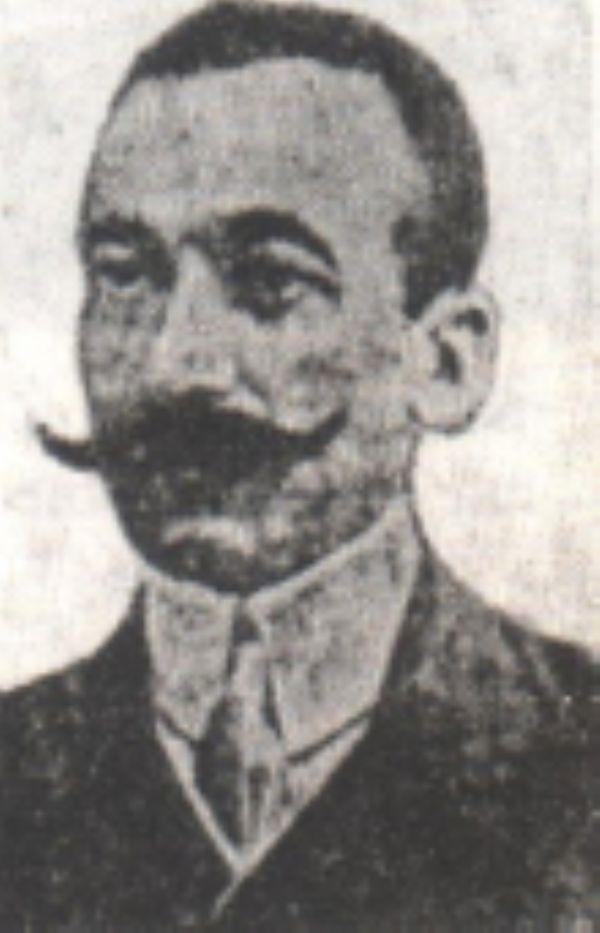The image is an old, slightly blurry black-and-white portrait of a Caucasian man with very short dark hair and a receding hairline, facing slightly to the left. His prominent right ear, cheek, and jawline are clearly visible, while the left side of his face is partially obscured. He has thick, black eyebrows and a very large, pointed, and curled mustache that extends beyond his face, covering his entire upper lip. His serious eyes stare solemnly ahead. The man is formally dressed in a dark jacket and a large white-collared shirt, possibly with a light gray tie, though the grayscale shading makes it difficult to discern. The rectangular image, which is taller than it is wide, may be an old photograph or a detailed pencil or charcoal drawing set against a gray background.